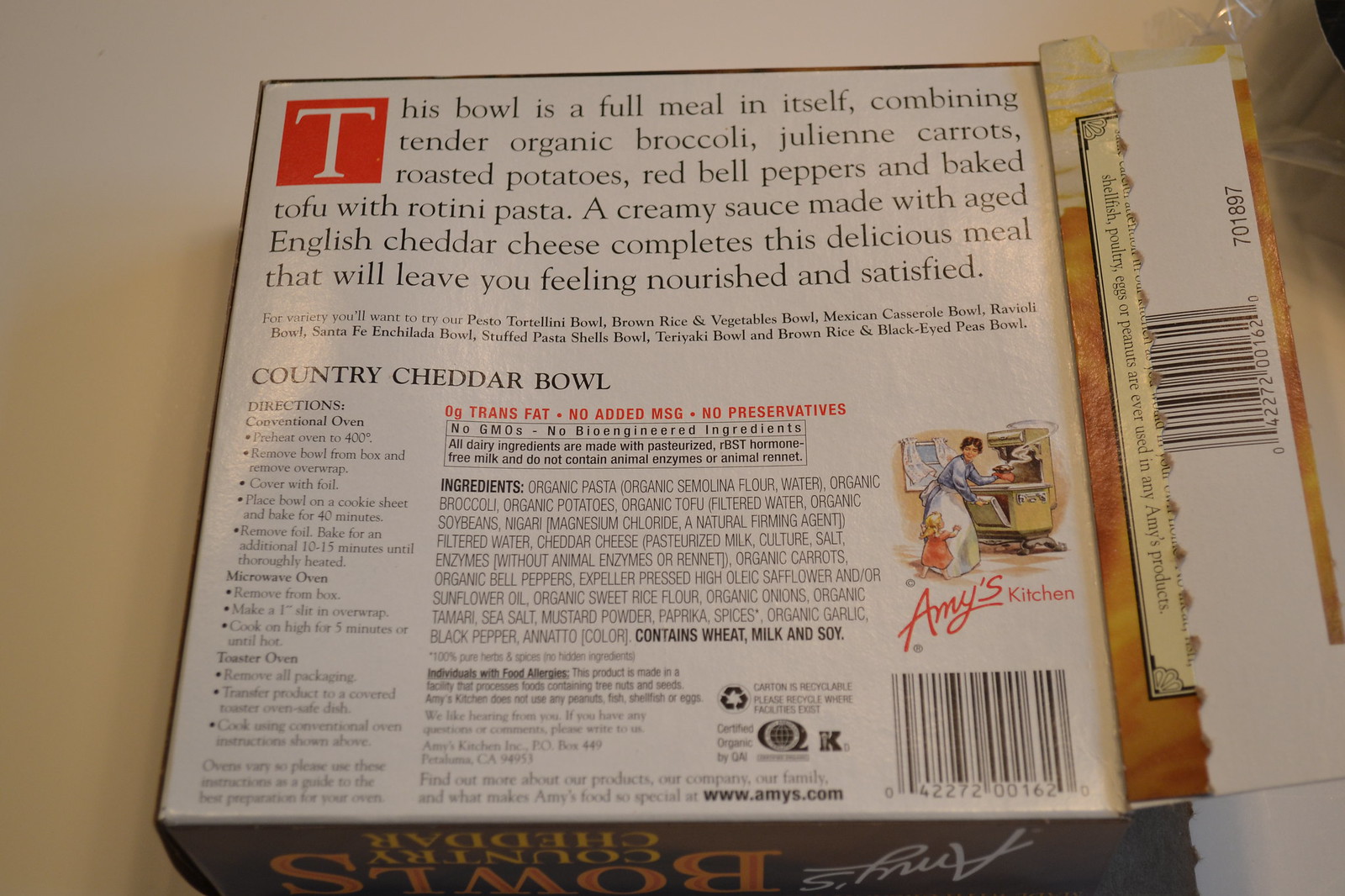This image showcases the back view of an Amy's Kitchen food package. The box features a vibrant color palette with shades of red, black, white, orange, and yellow. Prominently displayed at the top in a mostly black font is a detailed description of the meal. This Amy's Kitchen offering is a complete meal in a bowl, featuring tender organic broccoli, julienne carrots, roasted potatoes, red bell peppers, and baked tofu, all combined with rotini pasta. The dish is brought together with a creamy sauce made from aged English cheddar cheese, promising a satisfying and nourishing experience.

Beneath this description, the product name "Country Cheddar Bowl" is clearly stated in black font. The box also highlights key nutritional claims in red font, such as "zero grams trans fat," "no added MSG," and "no preservatives." Following this, a detailed ingredient list is provided, emphasizing that the product contains wheat, milk, and soy in bold black text.

Additionally, there is an evocative image on the back of the package depicting a woman with brown hair, dressed in a blue dress and white apron, standing by a window. She is seen opening an old-fashioned yellow stove, and in the background, a child with blonde hair and clad in red is visible, adding a touch of warmth and nostalgia to the packaging.